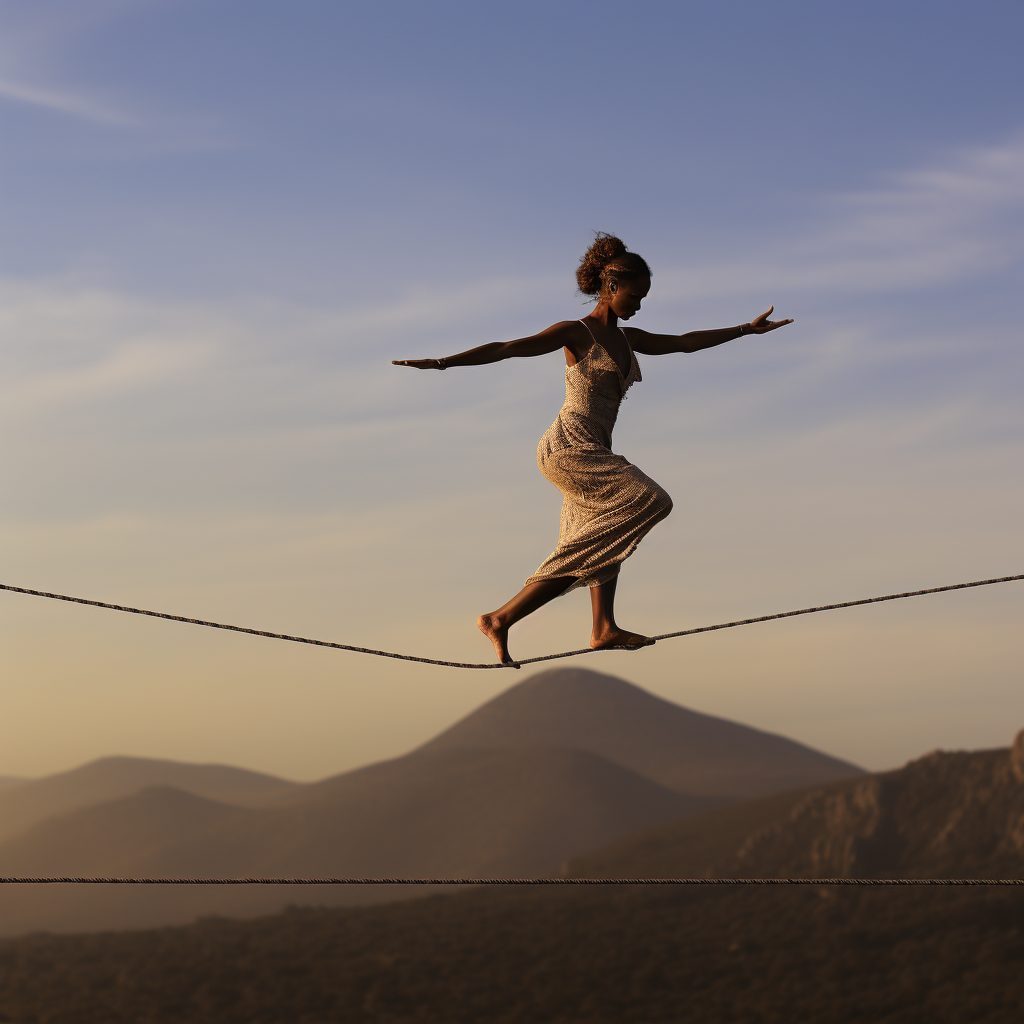In a serene landscape of rolling brown hills under a dusky sky, a woman with brown skin, possibly of African descent, is captured in an elegant act of balance on a tightrope. She dons a white, patterned spaghetti strap dress that softly flows with her movements, and her hair is secured in a neat ponytail or bun. With her knee bent toward the viewer, she extends her arms for balance—her front arm held palm up and the back arm palm down. Below her, another tightrope stretches across the scene, subtly slacked into a shallow V. The sky above the hills is a pale blue, hinting at sunset, with delicate wisps of clouds adding to the tranquil ambiance. She gazes down at her feet, embodying both grace and control, fully immersed in her precarious yet poised walk.